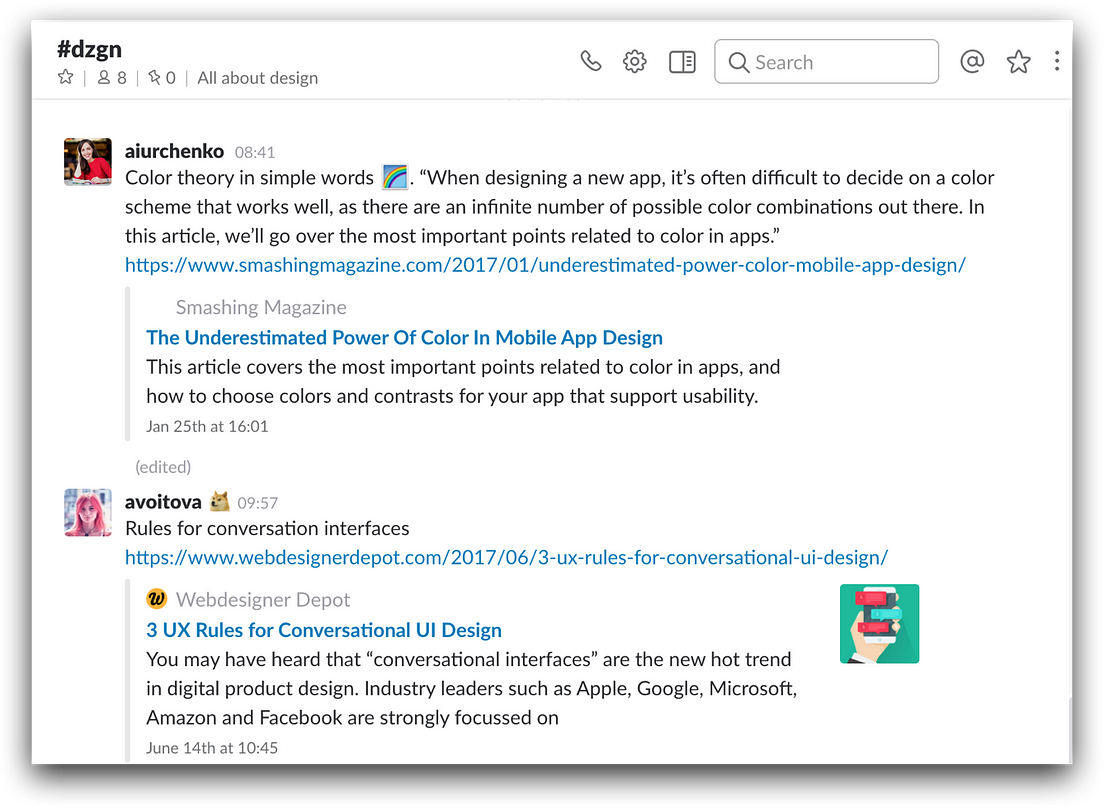### Slack Design Channel Overview

**Channel:** #DZGN  
**Description:** All about design  
**Members:** 8  
**Pinned Items:** 0  

---

#### Post 1 by Airchenko (08:41)

**Profile Picture:** Woman in a red shirt

**Title:** Color Theory in Simple Words

**Content:**  
> 📷 "When designing an app, it's often difficult to decide on a color scheme that works well as there are an infinite number of possible color combinations out there. This article will go over the most important points related to coloring apps."

**Link:** [The Underestimated Power of Color in Mobile App Design](https://www.smashingmagazine.com)  
**Source:** Smashing Magazine

**Description:**  
> "This article covers the most important points related to coloring apps and how to choose the colors and contrasts that support usability."

**Posted On:** Jan 25th at 16:01

---

#### Post 2 by Avoidtova (09:57)

**Profile Picture:** Woman with pink hair, Doge emoji

**Title:** Rules for Conversation Interfaces

**Content:**  
**Link:** [Three UX Rules for Conversational UI Design](https://www.webdesignerdepot.com)  
**Source:** Web Designer Depot

**Description:**  
> "You may have heard that conversational interfaces are the new hot trend in digital product design. Industry leaders such as Apple, Google, Microsoft, Amazon, and Facebook are strongly focused on it."

**Posted On:** June 14th at 10:45

---

**Interface Elements:**

- **Top Left:** Channel name (#DZGN)
- **Top Right:**  
  - Icons for iPhone, settings (gear icon), and a square with lines (possibly for messages or documents).
  - Search bar (magnifying glass) with "Search" placeholder.
  - Additional icons: app symbol, star, and three vertical dots (settings or more options).

This screenshot serves as a succinct glimpse into the Slack channel focused on design, illustrating active posts and key tools accessible to members.